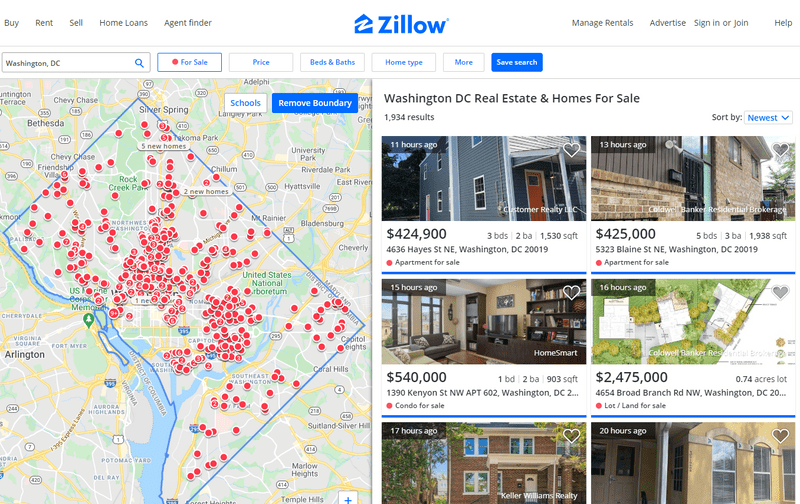The image is a screenshot of the Zillow real estate website's main page interface. At the center of the page is Zillow's iconic house logo featuring a lightning bolt-shaped 'Z' and the brand name 'Zillow' in blue. 

To the left of the logo, there is a navigation menu listing options: 'Buy,' 'Rent,' 'Sell,' 'Home Loans,' and 'Agent Finder.' On the right side of the logo, there are additional options including 'Manage Rentals,' 'Advertise,' 'Sign In or Join,' and 'Help.'

Below the logo and navigation menu, the website's main search functionality is displayed. A large search bar contains the pre-filled text "Washington DC," accompanied by various filtering options like 'For Sale,' 'Price,' 'Beds & Baths,' 'Home Type,' 'More,' and 'Save Search.' Notably, the 'For Sale' option is selected, indicated by a red dot and blue outline, while the 'Save Search' button is prominently solid blue with white text.

Under the search bar, there is an interactive map highlighting the Washington DC area, marked with numerous red dots indicating properties for sale in regions such as Bethesda, Chevy Chase, Silver Spring, Hyattsville, and Arlington, Virginia. Additional map features include options for displaying local schools and removing boundary restrictions.

To the right of the map, the number of real estate listings is summarized with the text "Washington DC real estate and homes for sale, 1,934 results." Directly beneath this text, there is a sorting dropdown menu labeled 'Sort by: Newest,' highlighted in blue with a down arrow to access other sorting options like price order.

At the bottom of the screenshot, preview images of the six most recently listed homes are displayed, each with a small banner indicating the time since listing: "11 hours ago," "13 hours ago," "15 hours ago," and "16 hours ago," respectively. This section provides a quick view of the latest real estate opportunities in Washington DC.